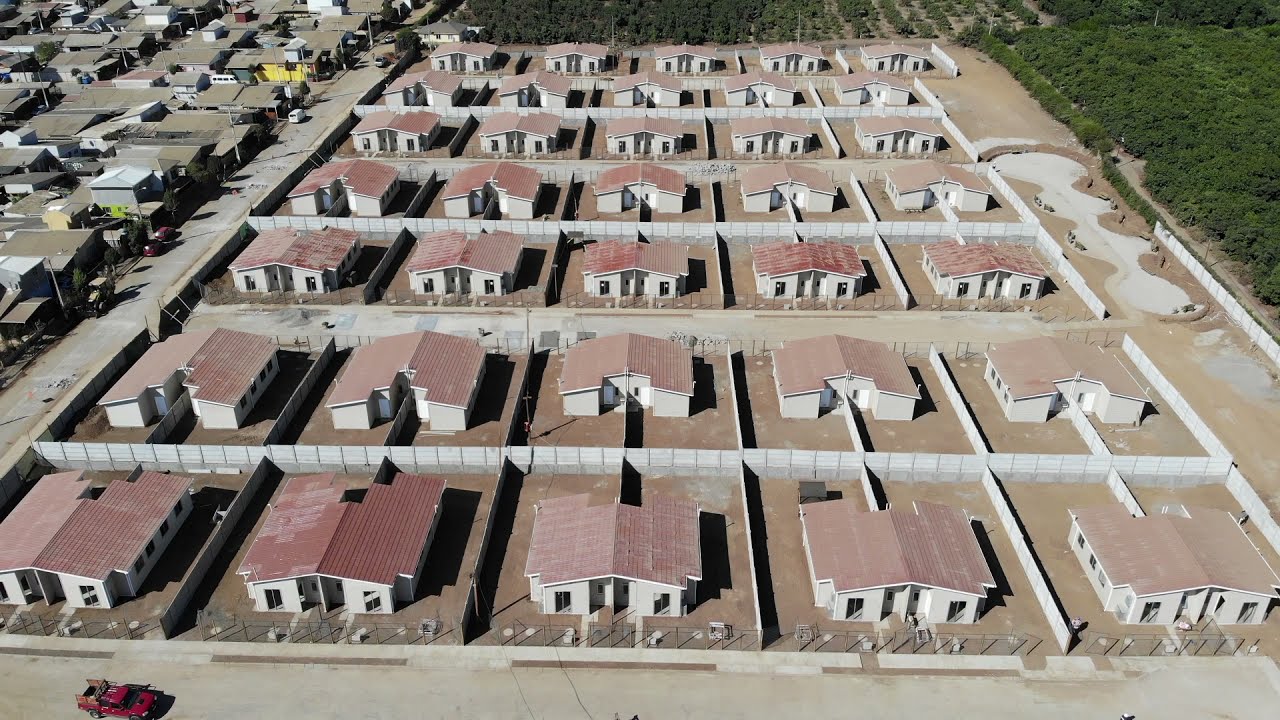The aerial image depicts a newly constructed housing development featuring a block of uniformly designed homes, set in a large neighborhood or complex. The houses are arranged in seven rows of five columns, totaling 35 identical homes, each situated on square plots with bare dirt yards indicating no landscaping has been done. These symmetrical structures share a consistent design with cream-colored exteriors, red-tiled roofs, central doors, and windows on both sides. The overall construction phase suggests the homes are uninhabited, with no visible people or possessions. The upper right-hand corner of the image shows green grass or trees, while the upper left-hand corner contains other densely packed houses, adding context to the neighborhood's setting.